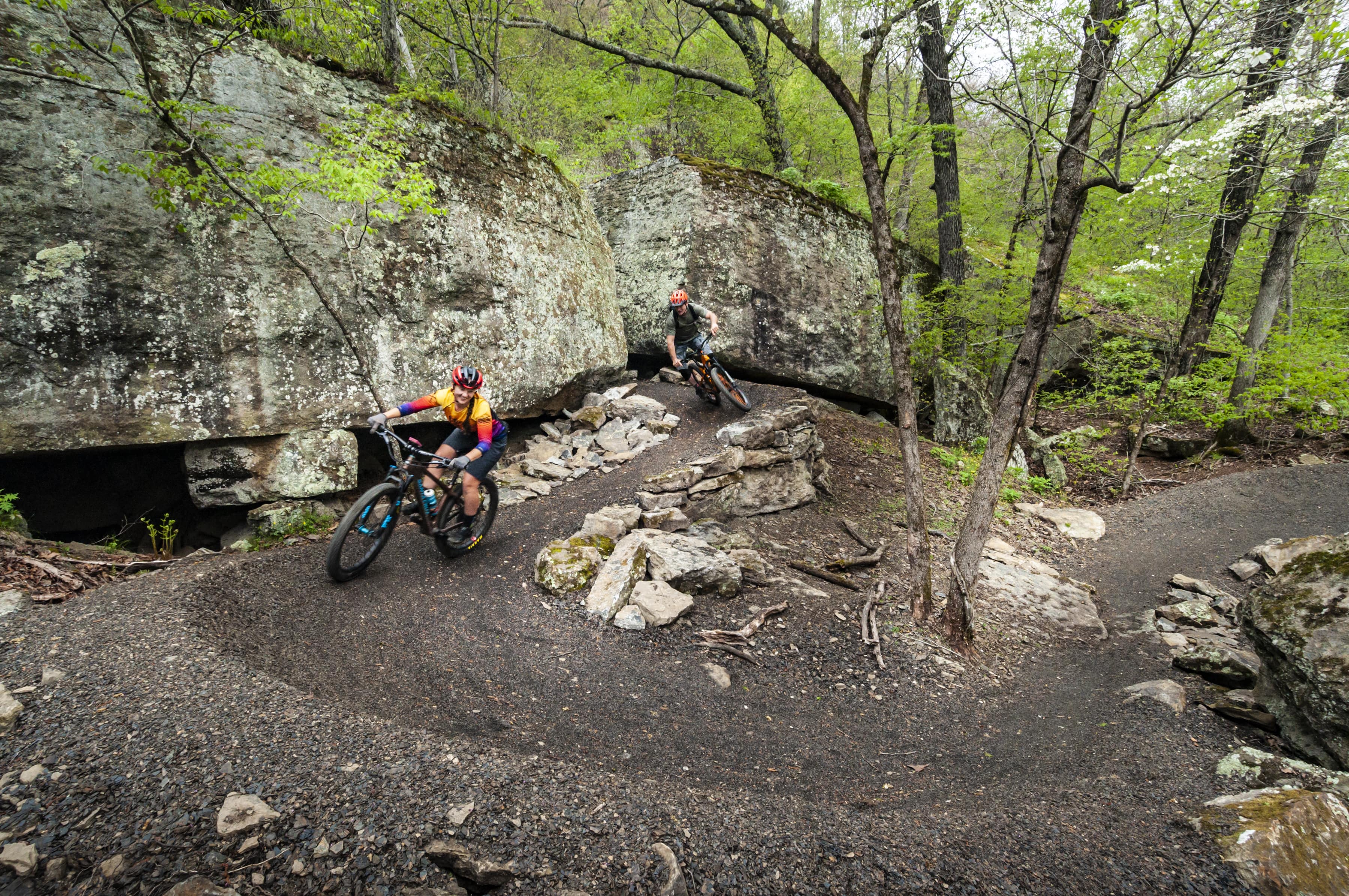The image captures two young bikers navigating a narrow, winding dirt path that snakes through a forested area, wrapping around trees and rocks in a horseshoe pattern before curving off-screen to the right. The trail, which is clear-cut yet surrounded by rough terrain featuring large rocks and dense foliage, suggests an adventurous, skilled ride. They appear to have emerged from a small canyon-like gap between two towering rocks. Both riders are dressed in professional cycling attire and helmets, emphasizing the necessity of safety gear. The rider in front sports a vivid outfit in yellow, red, and blue, while the rider behind wears less bright attire. Despite the challenging path, the young bikers seem to be enjoying the ride, suggesting a sense of thrill and accomplishment in this outdoor setting.